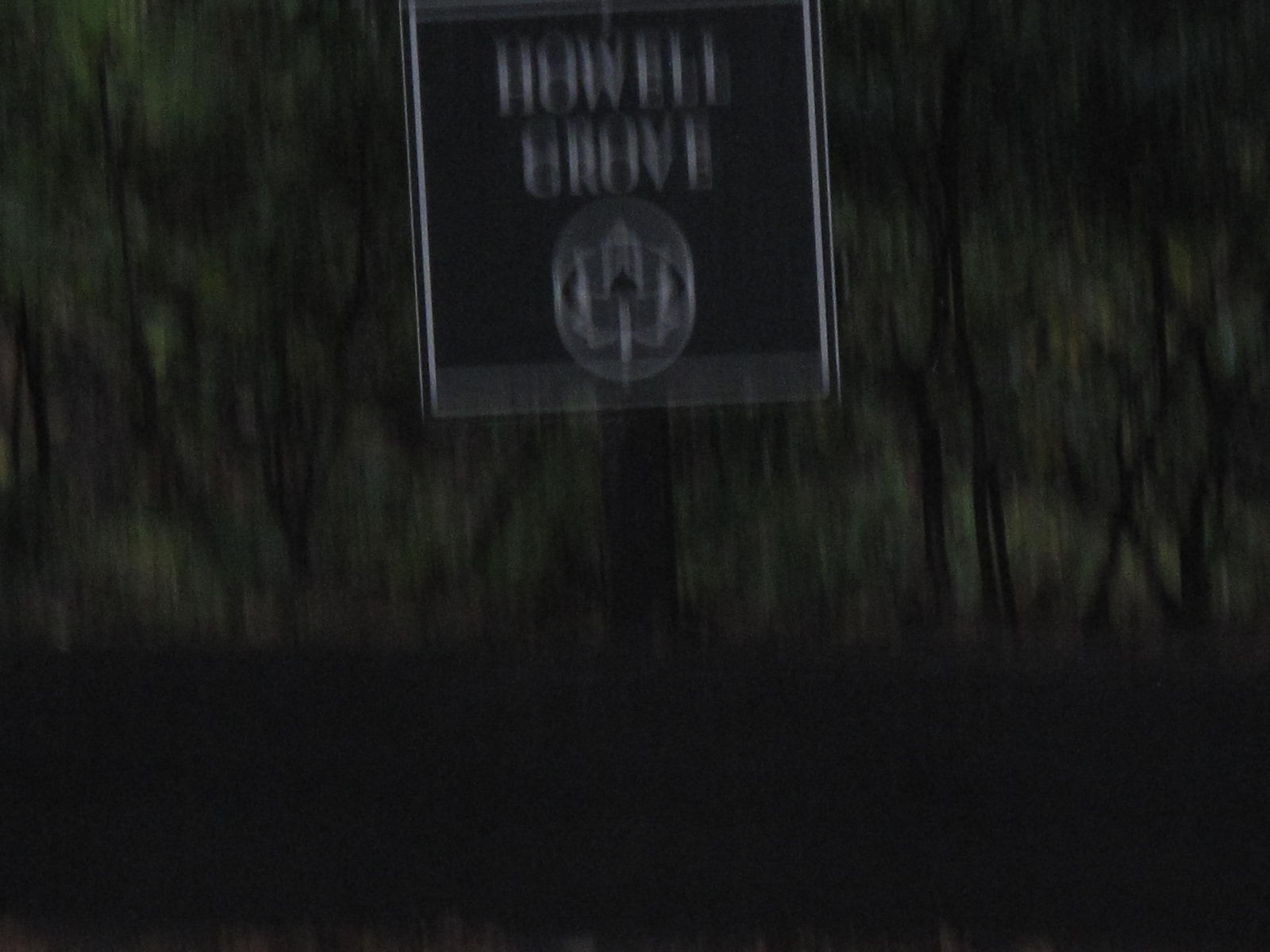The image depicts a nighttime, outdoor scene with a blurry, black, rectangular street sign that has a white border. The sign appears to say "Howell Grove" at the top with elongated, shaky letters due to camera movement. Below this text, there is a circle containing a white maple leaf symbol. The sign seems to be attached to a black pole. The dark background is indistinct but suggests the presence of trees or branches. The overall photo is very dark and shaky, contributing to the ghostly, wavy appearance and making other details difficult to discern.